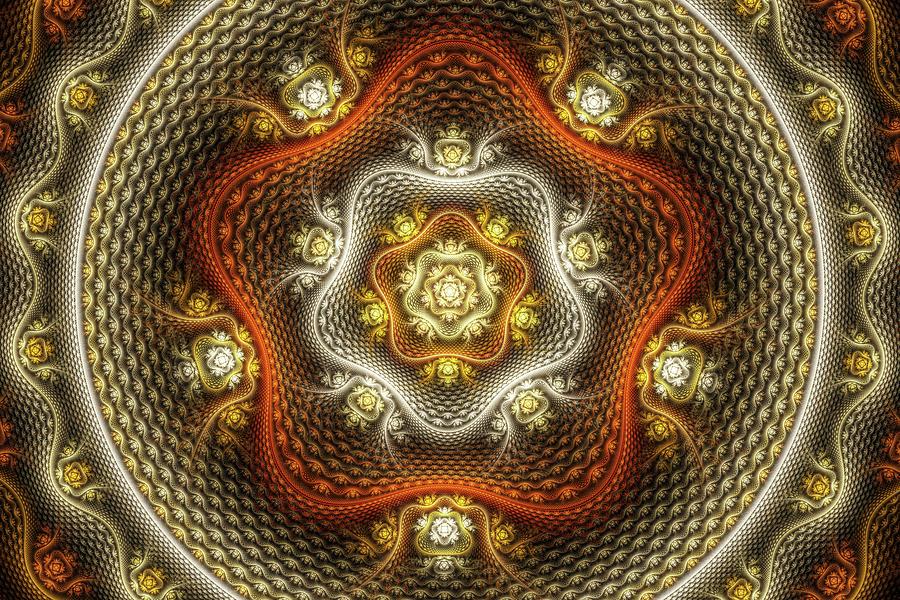The image appears to be an intricate, computer-generated or painted design with a striking, flower-like composition that plays with optical illusions. At the center, there's a star-shaped geometric design in yellow, surrounded by progressively larger and similar floral patterns in an array of colors, including yellow, white, orange, red, and gold. The design radiates outward, each layer growing in size and complexity. The outer layers feature a red floral motif, eventually transitioning into a large circular area detailed with tiny flower patterns and an elaborate, basket-like overall appearance. The edge of the design is bordered by wavy lines and intricate patterns, including swirls, dots, and miniature crowns, adding to the ornate nature. The image combines browns, whites, golds, yellows, and reds, creating a dynamic visual effect that makes the shapes appear as if they're either emerging from or receding into the background.